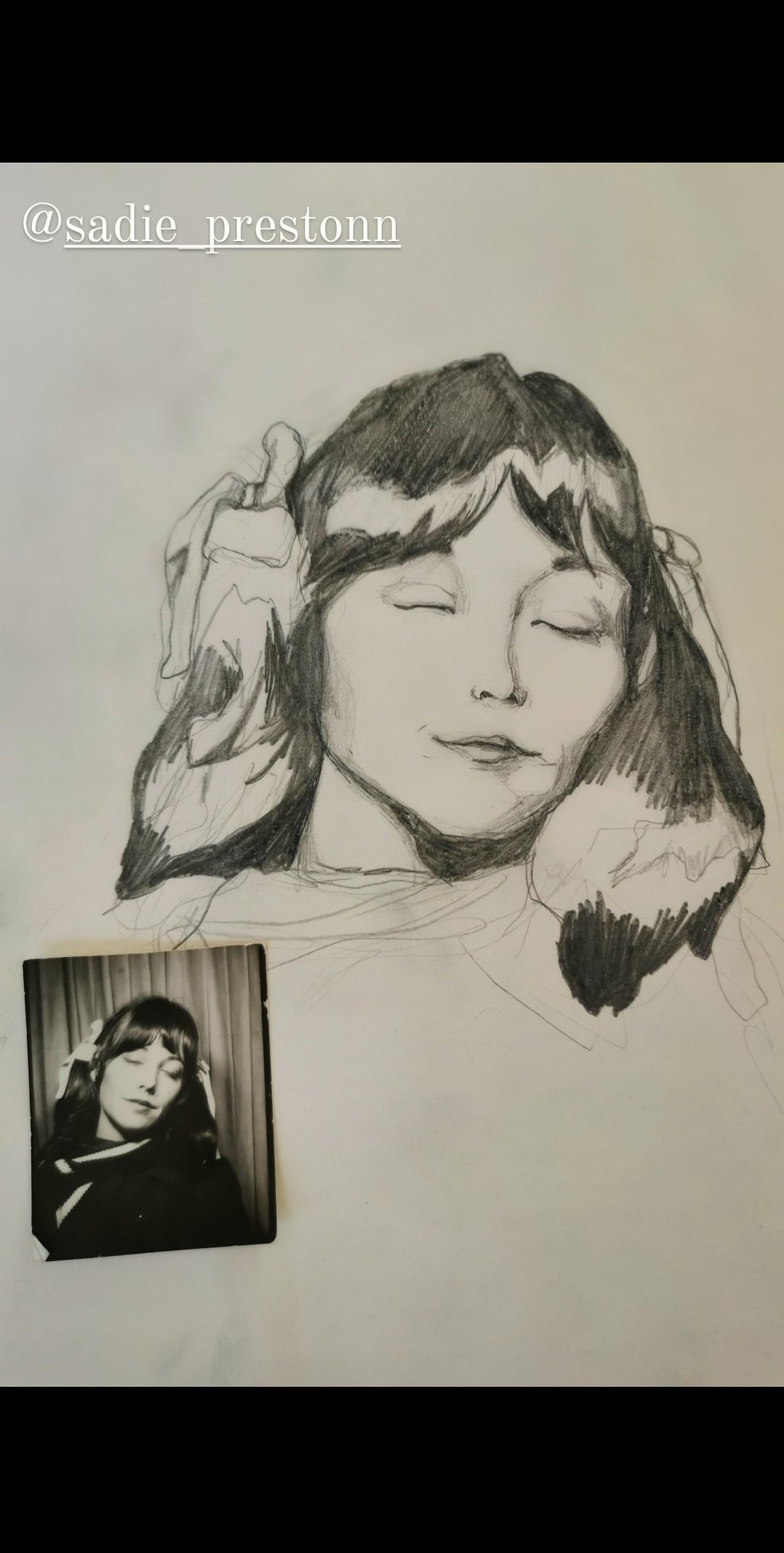**Caption:**

Screenshot of a social media profile belonging to @Sadie_Prestonn. The profile features a hand-drawn portrait of a woman with flowing brown-black hair, adorned with white cloth elements, cascading past her shoulders. In the bottom left corner, there is a real-life photograph of the same woman, showcasing brown hair with decorative ties woven into it.